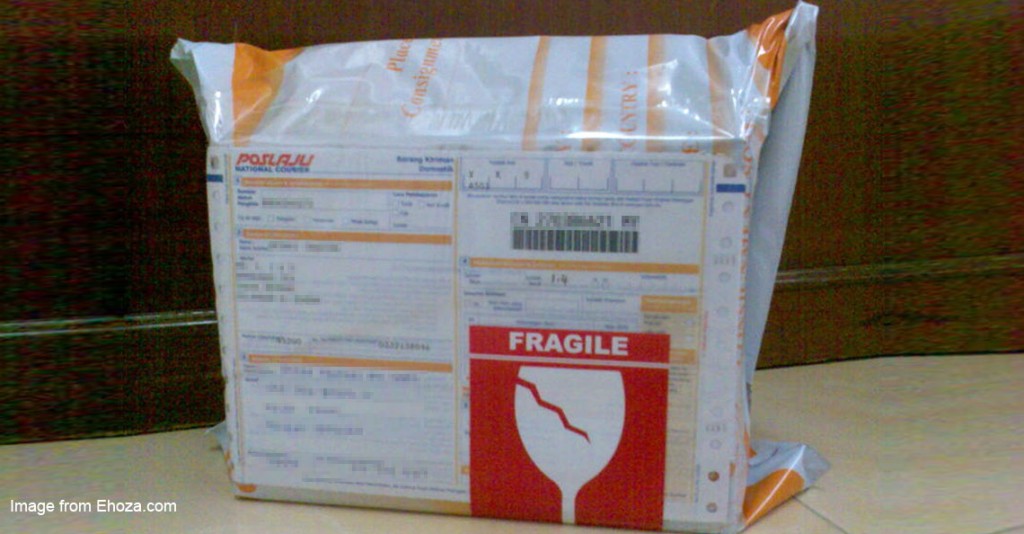The photorealistic image depicts a package wrapped in white and yellow plastic, resting on a tan-colored floor. The package bears a red "fragile" sticker with a cartoon depiction of a shattered glass in white, located prominently on the bottom right-hand side of the shipping label. The shipping label itself features orange and blue text, and while it includes shipping details, they are largely illegible. The top left corner of the package displays the shipping company name "POSLAJU" in red letters. The background of the image is dark, occupying the top two-thirds of the frame behind the package. In the bottom left-hand corner of the image, the phrase "image from ehoza.com" appears in white text. The scene is well-lit, capturing the details of the package and its surroundings with clarity.